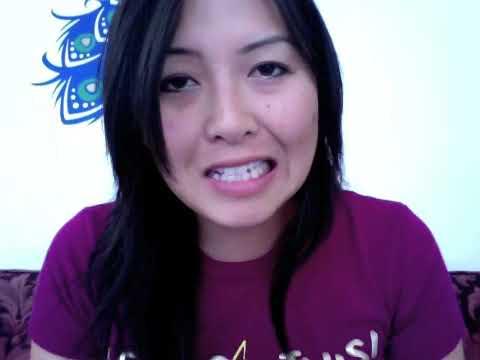This indoor image captures a well-lit, white-walled room. Prominently in the center foreground stands a young woman with long, straight, dark brown hair, possibly of Asian descent. She is wearing a short-sleeved, deep fuchsia shirt with the word "THIS" partially visible, with other letters obscured by her hair and gestures. She is looking directly at the camera, gesticulating with her hands raised. In the background, on the top right-hand side, a floating wooden shelf holds indistinct items, potentially including a vase and picture frames. On the left-hand side, there is a bookshelf filled with various books or media. Her head is positioned towards the top of the image, and her attire and positioning suggest she might be engaged in a video call or recording.